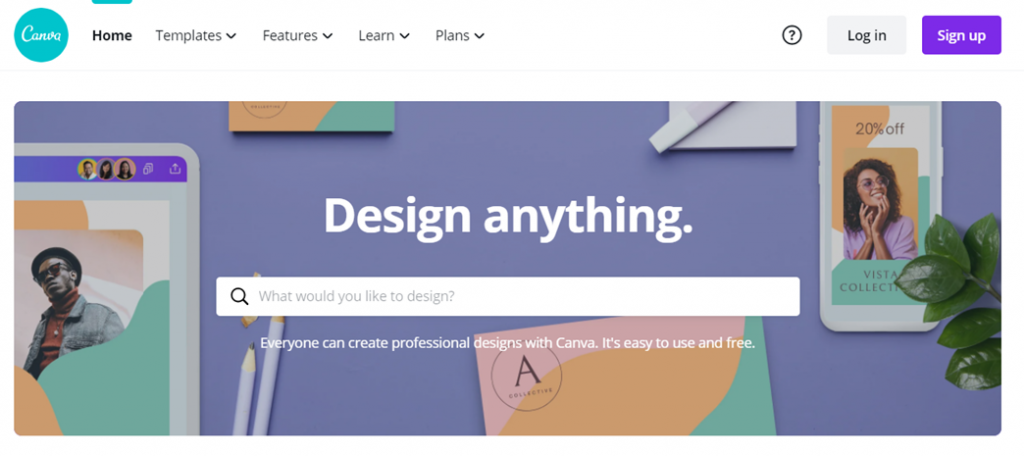The webpage header features several menu options including "Home," "Templates," "Features," "Canna," "Learn," and "Plans," each accompanied by dropdown menus. A black question mark icon appears next to these options, followed by "Log In" and "Sign Up," with the "Sign Up" button highlighted in purple.

Below the header, the main section of the page prominently displays the headline "Design Anything" in white text. To the left of the headline stands a man, and to the right, a woman. Centered between them is a white search bar. The background of this section is blue and is adorned with colorful objects including a pink piece of paper, an orange phone, and a green plant positioned to the right. Additionally, there are two white pencils on the left and an eraser at the top right corner of the page. An orange phone above the woman displays a banner reading "20% off."

A promotional message below the search bar reads, "Everyone can create professional designs with Canva. It's easy to use and free. What would you like to design?" Finally, a large black letter 'A' inside a black circle is subtly integrated into the middle-bottom background of the page.